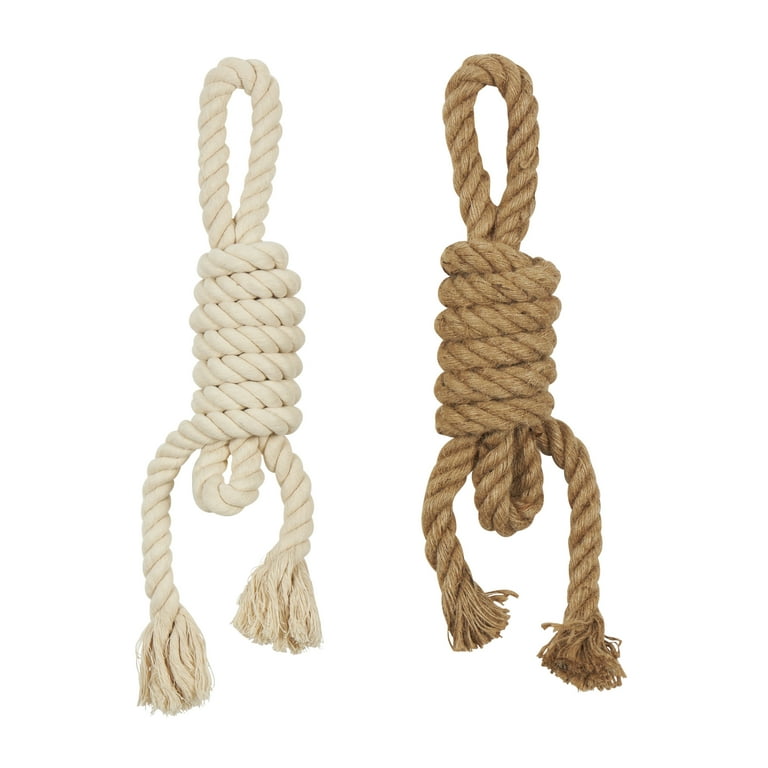This photo features two ropes tied into intricate knots against a clean white background. On the left side is a white rope, and on the right side, there is a darker beige traditional rope. Both ropes are tied into the same type of knot formation. Each rope showcases a large loop at the top that resembles a noose, followed by seven swirls or braids in the white rope and six in the beige rope, creating a cylindrical, twisted appearance. The middle section of each rope displays these swirls prominently, adding a braided texture. At the bottom, both ropes end in much smaller loops with fringed rope ends extending from each side. The knots are meticulously tied, demonstrating a proper method of securing the ropes, perhaps suggesting an advertisement showcasing the durability and quality of the ropes.